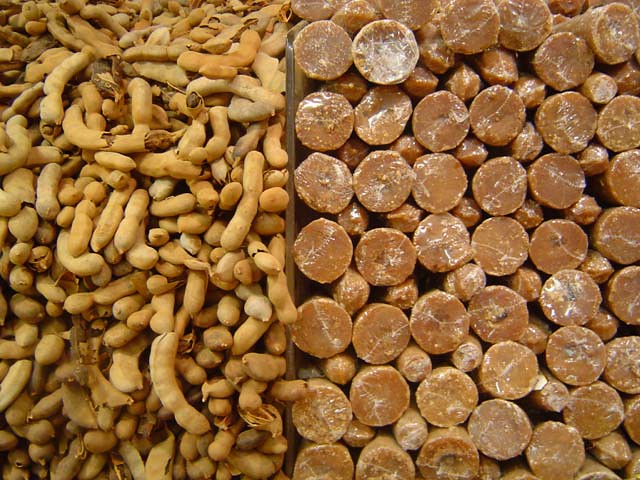The image is a horizontally aligned rectangular photograph divided into two vertical sections. The left-hand side features a variety of legumes, possibly peanuts, enclosed in light tan and beige pods. Some pods contain three or four lumps, while others are smaller, completely covering this portion of the image. Notably, a few of the pods have chipped shells, revealing a darker brown interior. On the right-hand side, there are medium brown, cylindrical objects stacked on top of each other, resembling candies, such as inverted Rolos. These objects have a peanut butter-like color with occasional white streaks. The image clearly separates the two categories with a distinct divider.